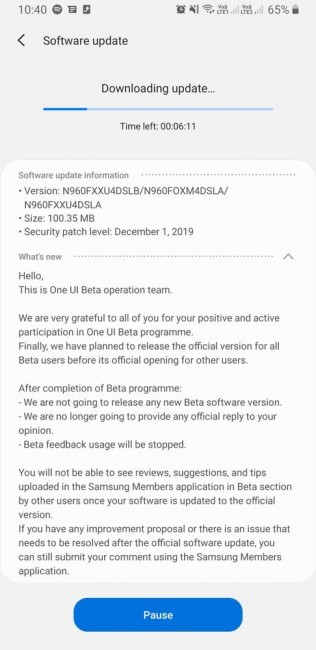In this screenshot, the gray header at the top displays a variety of status information. In the upper left corner, the time reads 10:40. On the upper right side, there are several icons: an alarm clock, Wi-Fi signal strength indicating it is on, a sound icon showing it is muted, LTE signal, and a battery icon indicating 65% remaining.

Beneath the header, on the left side, there is a prompt for a software update signified by an arrow pointing left. Below this prompt, text informs the user of an ongoing download indicated by the phrase "Downloading update" accompanied by a blue horizontal progress bar. The remaining time for the download is specified as 6 minutes and 11 seconds.

Against a white background further down, detailed information about the software update is provided. The update version is listed as N960FXXU4DSLB, with a total size of 100.35 MB. The security patch level is dated December 1st, 2019. 

At the bottom, a message from the One Beta Operation Team reads: "Hello, this is One Beta Operation Team. We are grateful to all of you for your positive and active participation in the One UI Beta Program.”